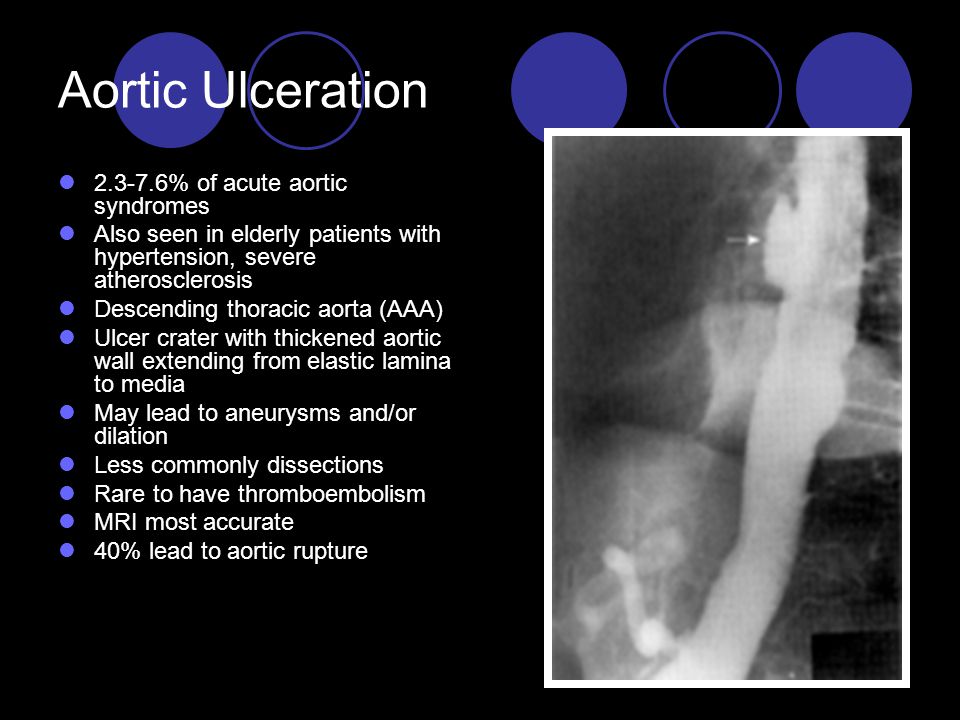The image prominently displays the title "Aortic Ulceration" in white text at the top left corner, superimposed on a black background. Just beneath this title, additional detailed information is provided in white text, each statement marked by a small blue dot. The text reads: "2.3 to 7.6% of acute aortic syndromes. Also seen in elderly patients with hypertension, severe atherosclerosis, descending thoracic aorta, AAA. Ulcer crater with thickened aortic wall extending from elastic lamina to media. May lead to aneurysms and/or dilation. Less commonly dissections. Rare to have thromboembolism. MRI most accurate. 40% lead to aortic rupture."

The right side of the image features an x-ray that highlights the aorta, with a specific focus on the ulceration. The x-ray, adorned with an arrow pointing to the ulceration, depicts a large vessel running down the center of the image with a notable bulge, indicative of the aortic ulcer. Blue dots and outlined circles accentuate the background, contributing to the visual focus on the critical areas of interest. The overall layout effectively combines visual and textual information to document the medical condition in detail, emphasizing the urgency and importance of accurate diagnosis and treatment.